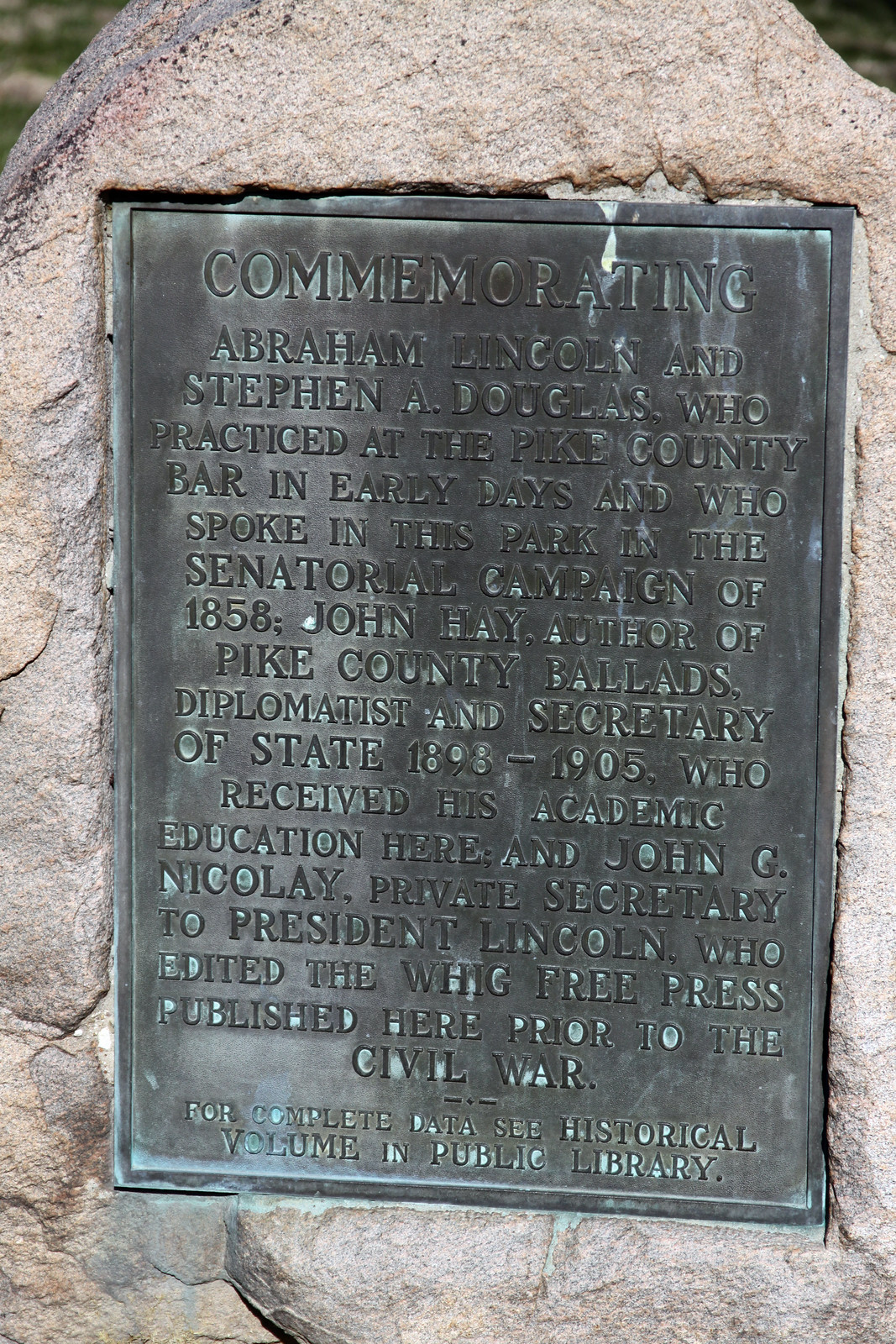The photograph, captured in portrait orientation, showcases a bronze commemorative plaque set into a large, oval, beige stone. The background setting is outdoors. The plaque, which has a weathered and green-tinged surface, bears raised, centered text that is difficult to read due to its aged condition. At the very top, in the largest font, is the word "COMMERMORATING." Below this, the plaque honors Abraham Lincoln and Stephen A. Douglas, mentioning their practice at the Pike County Bar and their speeches in the park during the 1858 senatorial campaign. It also commemorates John Hay, author of "Pike County Ballads" and Secretary of State from 1898 to 1905, who was educated in the area, and John G. Nicolay, private secretary to President Lincoln and editor of the Whig Free Press before the Civil War. The plaque concludes with a note directing readers to a historical volume in the public library for more information. The plaque is recessed slightly into the stone, with the text's difficulty exacerbated by its weathered letters.